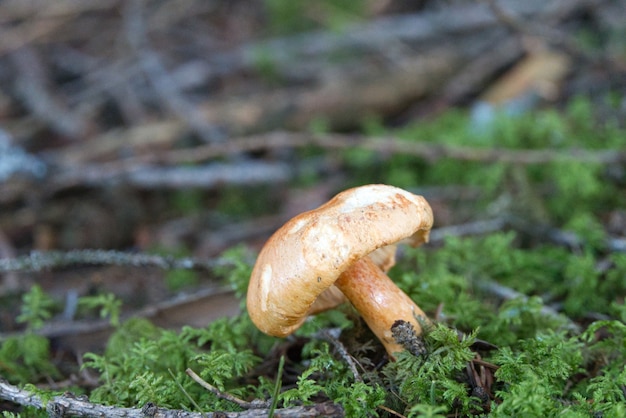In this close-up photograph set in a forest, a delicate mushroom with a white cap tinged with light brown stands out as it leans to the left, growing from the mossy forest floor. The mushroom is small and features a lighter underside with subtle striping. Nestled in the moss surrounding the mushroom is a tiny pine cone and several scattered twigs. The moss showcases intricate details like tiny leaves, adding texture to the scene. The background is softly blurred, revealing an array of sticks and branches in hues of grays and browns, creating a serene forest ambiance. The main colors highlighted in the image include the yellowish-brown of the mushroom, the dark green of the moss, and light gray-brown of the twigs. The overall composition draws rich attention to the natural beauty of the mushroom and its surroundings, captured effortlessly from a low angle.